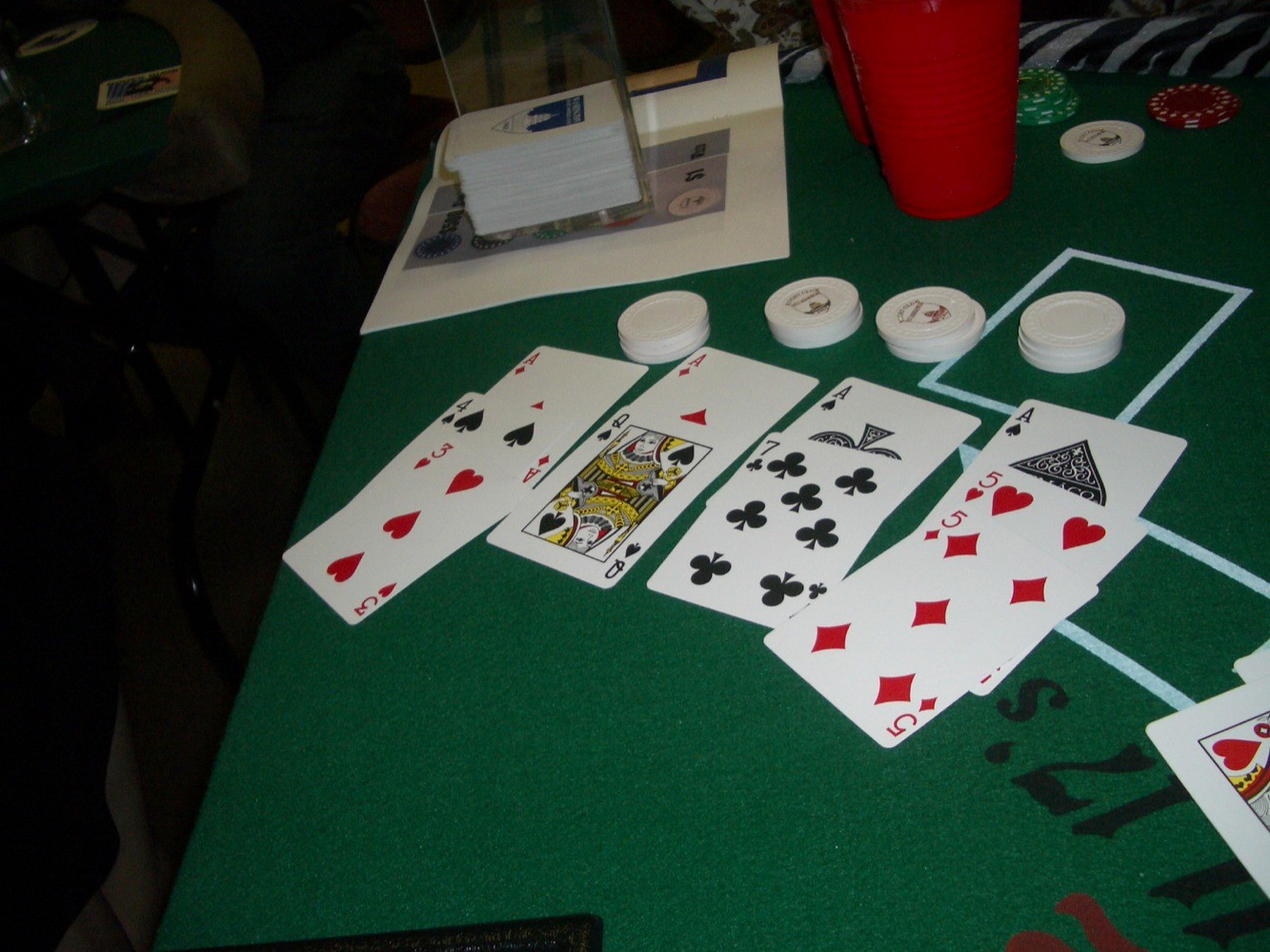The image showcases a dynamic poker game setup with a focus on a green felt poker table, predominantly on the right-hand side. The table is adorned with various elements that highlight an ongoing game. Two red Solo cups are placed at the top of the table, beside a scattered assortment of poker chips in green, red, and white. Additionally, there are neatly stacked white poker chips arranged in a curved pattern.

Several columns of playing cards are laid out across the table: 
- The first column features the 3 of Hearts atop the 4 of Clubs, which is atop an Ace of Diamonds.
- The second column displays the Queen of Spades over an Ace of Diamonds.
- The third column has the 7 of Clubs on an Ace of Diamonds.
- The fourth column shows the 5 of Diamonds on the 5 of Hearts, which is on an Ace of Spades.

On the left side of the table, which appears to be the dark side of the image, another half-poker table forms a half-circle shape, surrounded by various chairs. An open book, lying halfway off the table, hints at either game references or casual reading. Adjacent to the book, a clear plastic container holds additional playing cards. The backs of these cards feature a blue and white design with a distinctive white pyramid at the top.